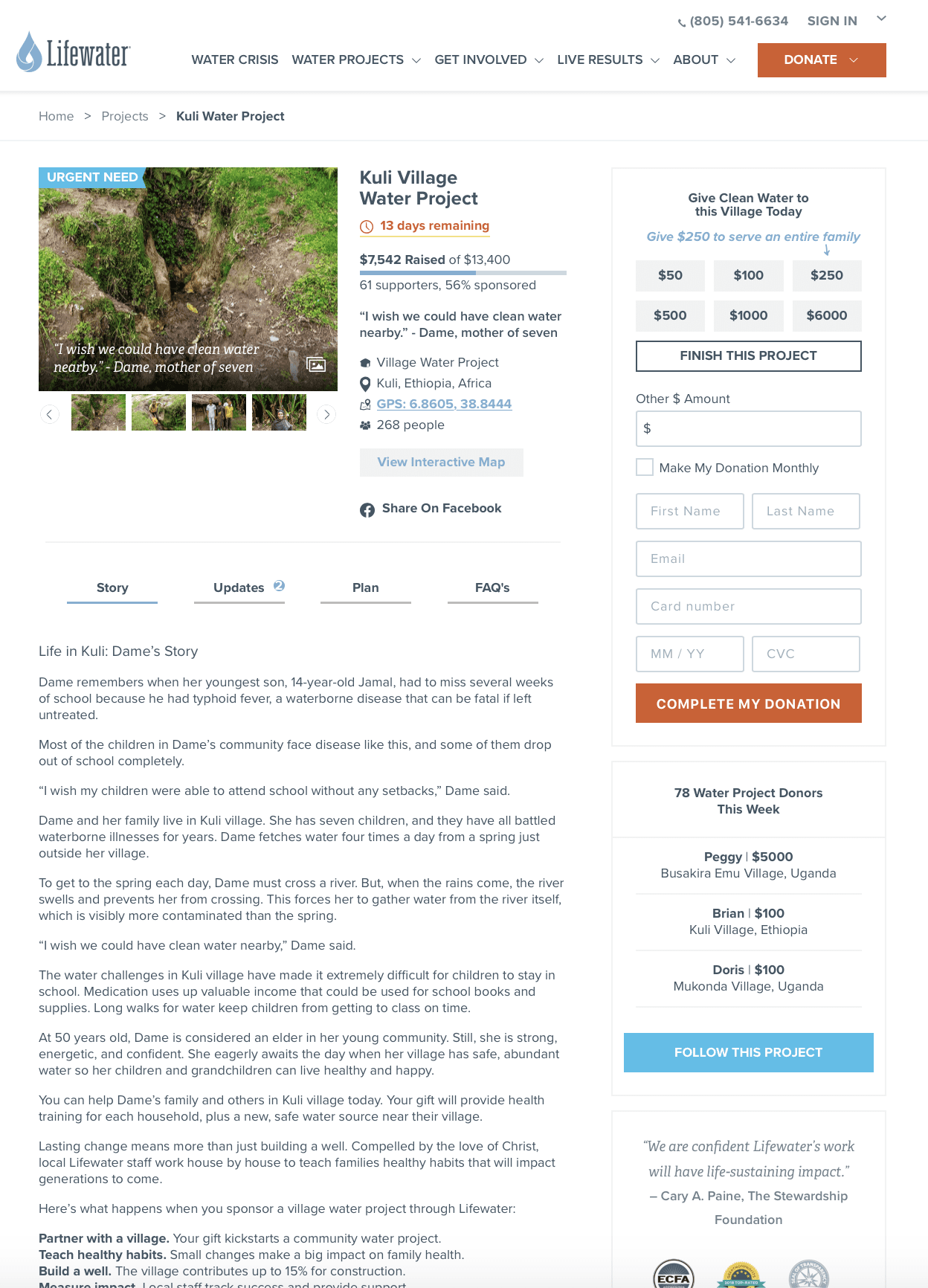This image is a detailed screenshot of a website dedicated to a water relief project named "Life Water." The header of the website features navigational tabs including "Water Crisis," "Water Projects," "Get Involved," "Live Results," "About," and a prominent "Donate" button.

To the left side of the screenshot, under the "Home Projects" section, there is a specific focus on the "Coulee Water Project." Beneath this, the title "Coulee Village Water Project" is displayed alongside a photo of some growing plants. Accompanying the image is a poignant quote: "I wish we could have clean water nearby," attributed to a pixelated name, identifying the speaker as a "Mother of Seven."

The project status is detailed to the right of this section, with a countdown indicating that 13 days remain for the campaign. The progress bar shows that $7,542 have been raised out of a $13,400 goal, marking the project as 55% sponsored with the support of 61 donors.

Below this, a set of buttons labeled "Story," "Updates," "Plan," and "FAQs" provide additional information about the project. A prominently titled story, "Life in Coulee: Tame Story," outlines life in the village and the impact of the water project.

The right side of the screenshot is dedicated to the donation process encouraging visitors to contribute with a call to action: "Give clean water to this village today."